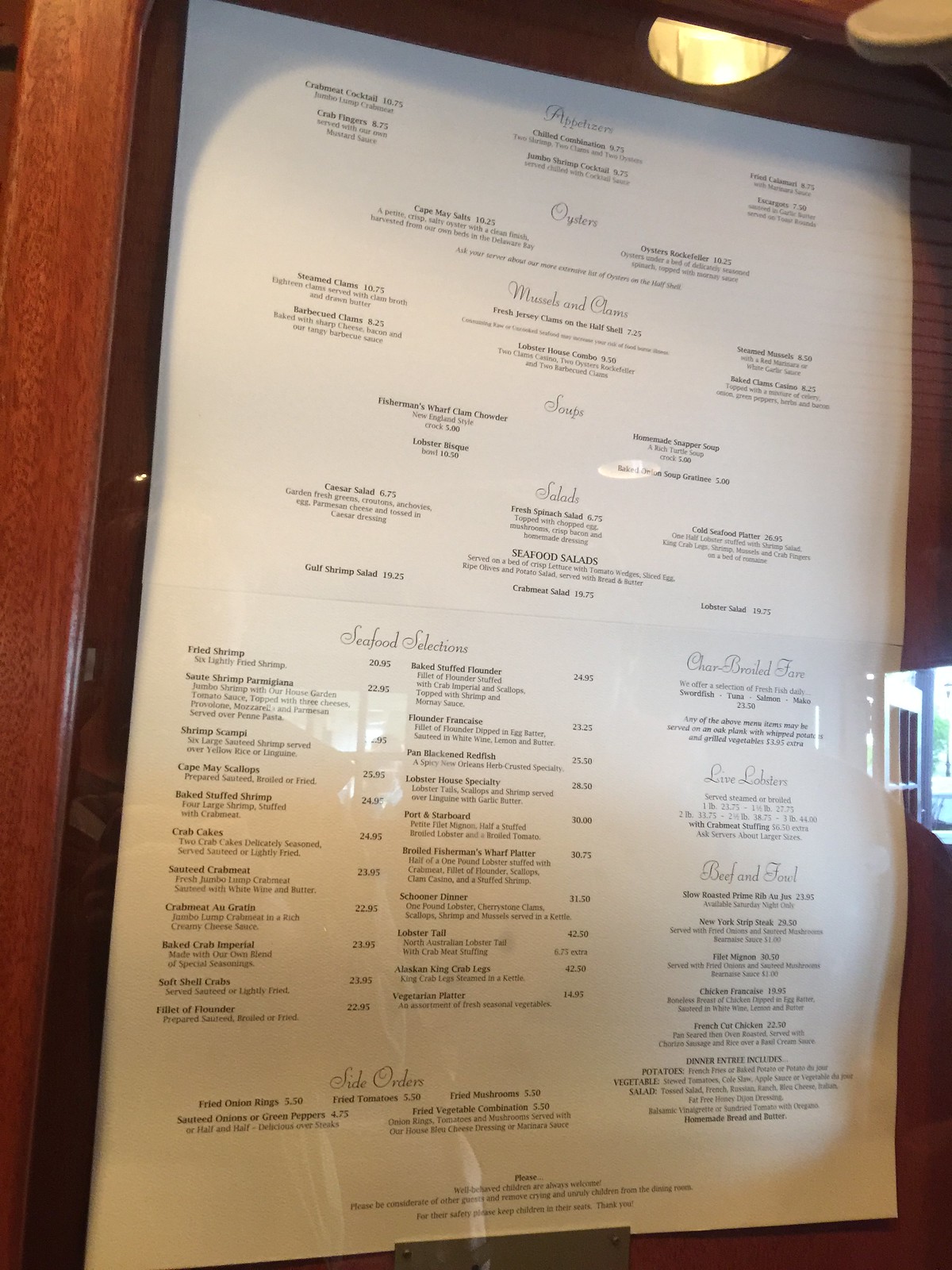The image features a framed menu placed on a dark brown table. The left side of the photo is predominantly occupied by the table's dark brown surface. The menu, which is more darkly framed in a similar brown hue, is positioned slightly right of center. The menu itself is square-shaped with a white interior paper displaying various menu options in extremely small text. 

At the top of the menu, horizontally listed items can be seen, gradually transitioning to the middle section. The bottom left section features two rows of vertically aligned menu items. On the right side of this section, there is a label accompanied by a few menu options, followed by another vertical row of menu items.

On the right side of the image, more of the brown table surface is visible. A blue light appears in the center-right of the image. The top of the image darkens further into an almost black shade, where a yellow light and a small part of a gray, flat-surfaced object can be found in the top right corner.